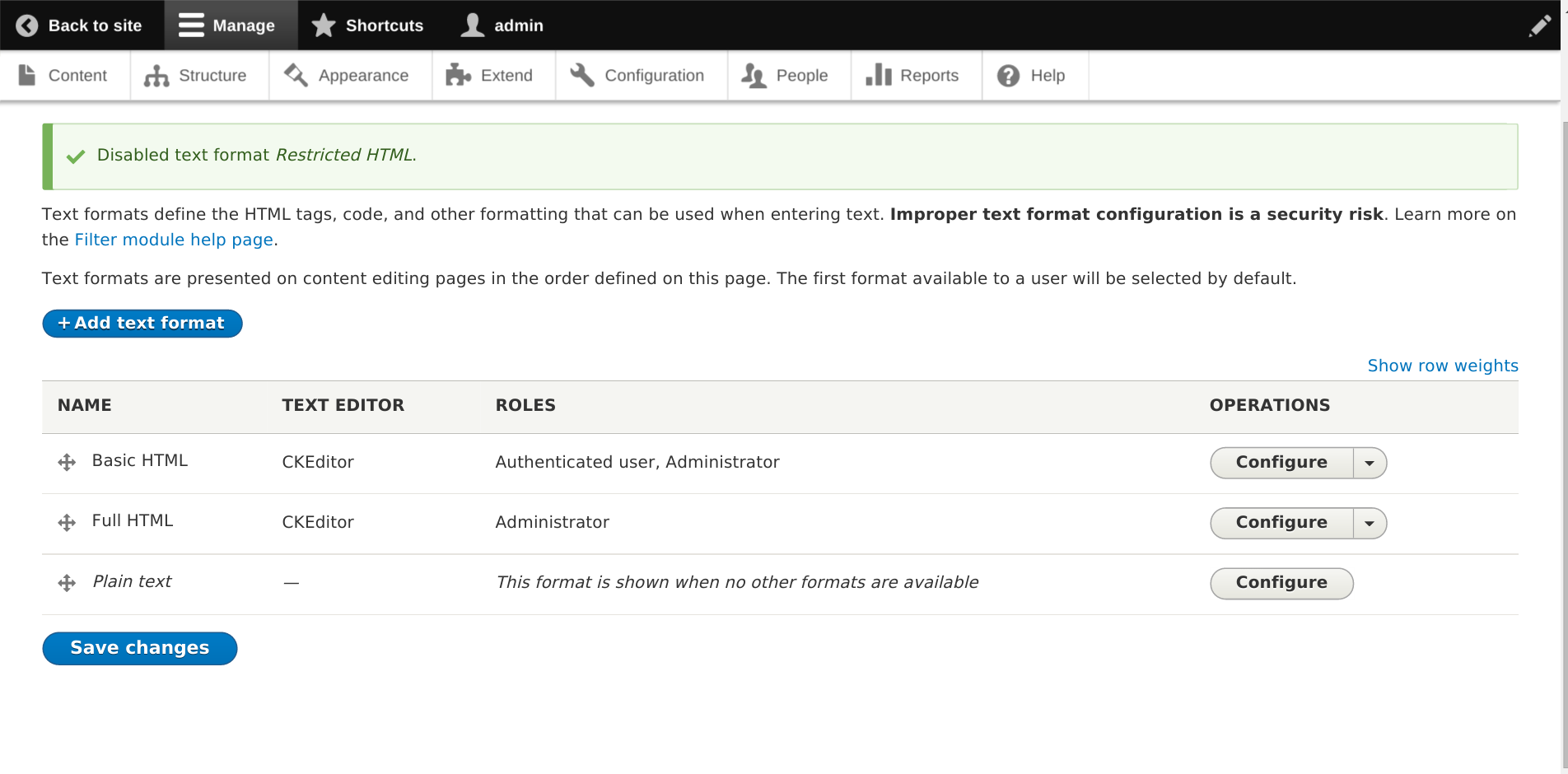Here's a detailed and cleaned-up caption for the image:

---

The screenshot depicts a web-based administrative interface primarily focused on managing text formats and HTML configurations. The user interface is simple and predominantly text-based, displayed against a white background with minimal graphical elements. 

At the top, there's a black header bar featuring navigation options in white text. On the upper left, a backwards arrow accompanied by "Back to site" is visible, suggesting a way to return to the main site. Adjacent to it are labels such as "Manage," leading into various administrative functions spread across this header.

Beneath the header, a row of clickable options is displayed in black print on a white background. These options include "Content," "Structure," "Appearance," "Extend," "Configuration," "People," "Reports," and "Help," each accompanied by simple, recognizable icons.

Subsequent to these options is a section highlighted with a pale blue background and bordered with green, containing a green check mark. The text here mentions "Disabled text format: Restricted HTML," emphasizing the importance of proper text format configuration to mitigate security risks. This section also directs the user to the "filter module help page" for further information.

In the middle of the interface, a blue-button featuring a white "+" symbol and the label "Add text format" stands out. Below this button is a table with a pale blue border, organizing content into columns labeled "Name," "Text Editor," "Roles," and "Operations."

The table lists three text formats:
- **Basic HTML**: Uses the "CKEditor" text editor and is available to both "Authenticated users" and "Administrators." It includes a "Configure" button for further customization.
- **Full HTML**: Also utilizes the "CKEditor" and is restricted to "Administrators," accompanied by its own "Configure" button.
- **Plain Text**: This format is depicted as a fallback option when no other formats are available.

Towards the bottom of the interface, a blue "Save changes" button provides the functionality to save any modifications made within this management panel.